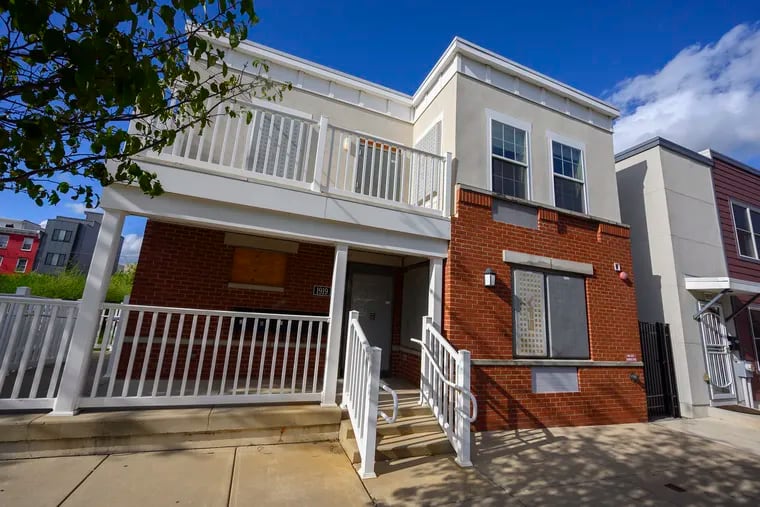The image depicts the front of an abandoned two-story building taken outside during the daytime, likely located in a city. The building's bottom half is made of red-orange brick, and the top half features a smooth, cream-white surface. The structure is very rectangular in shape and has a flat roof. The entrance is accessible via three stone steps that lead to a small covered patio or landing area with white wooden railings on either side. The first floor door and windows are boarded up with heavy, professionally-installed gray paneling, making it challenging to break through. Similarly, any accessible windows and doors on the second floor are also boarded up with the same type of paneling. However, two clear windows remain visible on the second floor, though they are difficult to access by hand. The second floor features a balcony with white railings supported by white wooden posts. In front of the building, there is a beige-colored sidewalk.

Adjacent to the building on the right, there is a similar-looking structure with red siding and white sections, separated by a narrow alleyway with a black gate. The neighbor appears inhabited, as its windows are not boarded up. In the far-off background on the left side, more buildings are visible, featuring gray and red facades. A green tree is seen on the left side of the image, and the sky above is bright blue with a few white clouds scattered around.